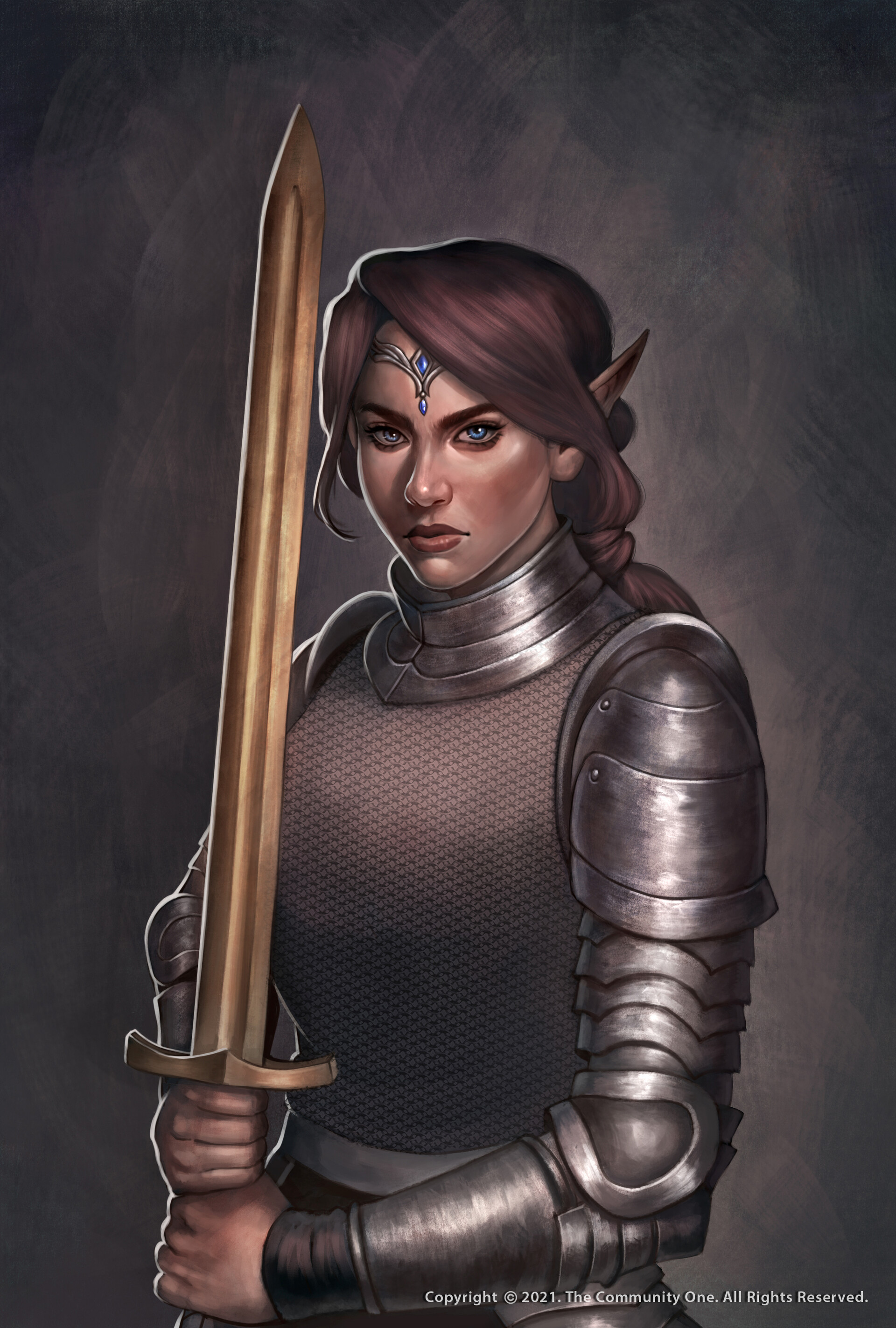This striking artistic image features a fantasy character drawn against a smoky, mystical background. The character is a female warrior, appearing to be an elf with pointed ears, a defining feature that sets her apart. She has long, brown hair with a reddish tint, styled into a ponytail with a few short layers framing her face. Her angled cheekbones, bright blue eyes, and makeup—including blush and lipstick—enhance her striking appearance. 

She wears a blue circlet around her forehead and full plate armor, visible from the waist up, with intricate iron fittings and armor extending down her arms and chest. She is depicted holding a gold sword with both hands, the blade extending from her waist to above her head. Her gaze is intense, directed straight at the viewer. 

In the bottom right corner, there is a discreet copyright notice in white text, stating: "© 2021. The community one. All rights reserved."